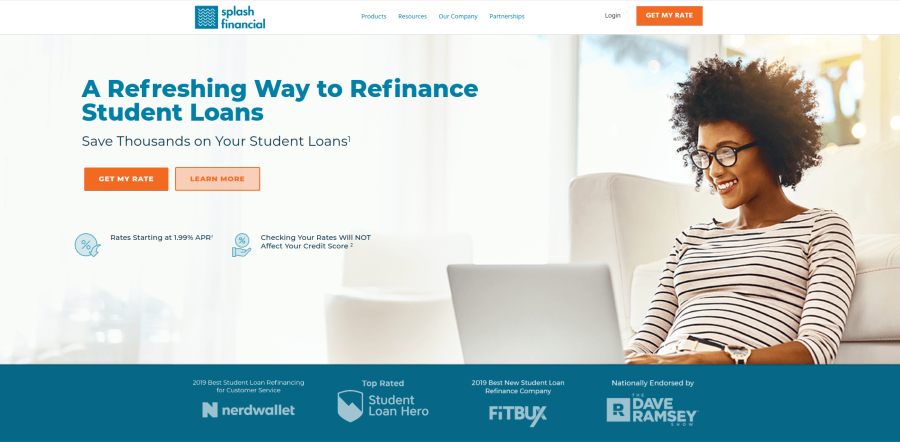The image is a screenshot of the Splash Financial website. In the upper left corner, there's a logo featuring a blue box with white squiggly lines. To the right of the logo, the company name "Splash Financial" is displayed. Centered in the header, there are navigation options in light blue font: "Products," "Resources," and "Company Partnerships." On the right side of the header, there's a white "Login" button, followed by an orange "Get My Rate" button in all caps.

Below the header, a welcoming image showcases a woman sitting on a white couch, smiling while using a computer. She is wearing glasses and a black-and-white striped shirt. To the left of this image, bold blue text reads, "A Refreshing Way to Refinance Student Loans." Beneath this, black text states, "Save Thousands on Your Student Loans." Below this text, there is another orange "Get My Rate" button, accompanied by a "Learn More" button to its right. At the bottom of this section, a small symbol is followed by the text, "Rates Start at 1.99% APR."